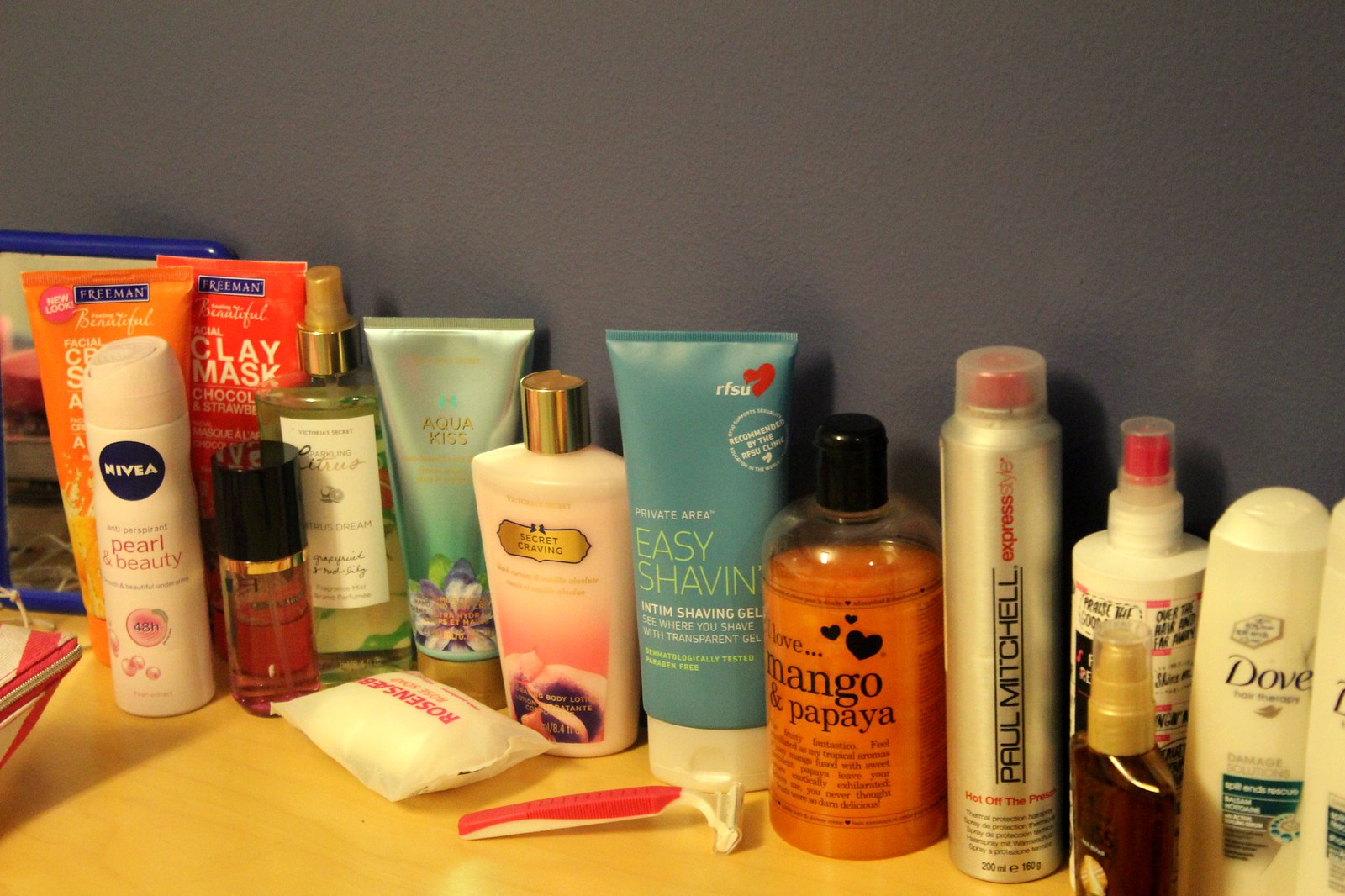Here is the cleaned-up and detailed caption:

The image features an array of bottled products set against a two-tone background, darkish gray at the top and an orange-yellow at the bottom. Starting from the left-hand side, near the bottom, there is a white and red item, difficult to identify. Next to it is a product outlined in thick blue, accented with red and gray. Moving right, there are orange and red containers, the red one labeled as a clay mask. In front of these containers, a white container with a black circle at the top bears the brand "Nivea" in white text, followed by indistinct smaller black text. Below, it boldly states "Pearl and Beauty" in red, with further small, unreadable text.

Following Nivea, a potential perfume bottle with a black cap appears, next to a clear bottle tinged with green, equipped with a spray top. Adjacent is a green container, golden at the bottom, depicting a flower with colors of white, purple, and green. In front of it lies a white packet adorned with pink writing. Nearby, another container with a gold cap seems to contain lotion. It features a gold banner with tiny writing at the top, transitioning into pink with a swirl of pink and purple at the base.

In front of this is a pink razor. Next to it stands a blue container with a red heart at the top right, white text, and circular inscriptions in white. It includes the phrase "easy shaving" in green, followed by more white and green text, too small to decipher. Further along, a clear container with a black top contains orange liquid, decorated with three hearts and unreadable text, except for "mango and papaya."

A spray can with a clear lid and a red and silver spray mechanism reads "Paul Mitchell" in black, flanked by fine lines above and below. Additional red and black text, too small to read, surrounds it. Another container in white, capped in red with a clear cover, is partially obscured by a tan to brown bottle. Finally, two identical bottles displaying the brand "Dove" complete the scene.